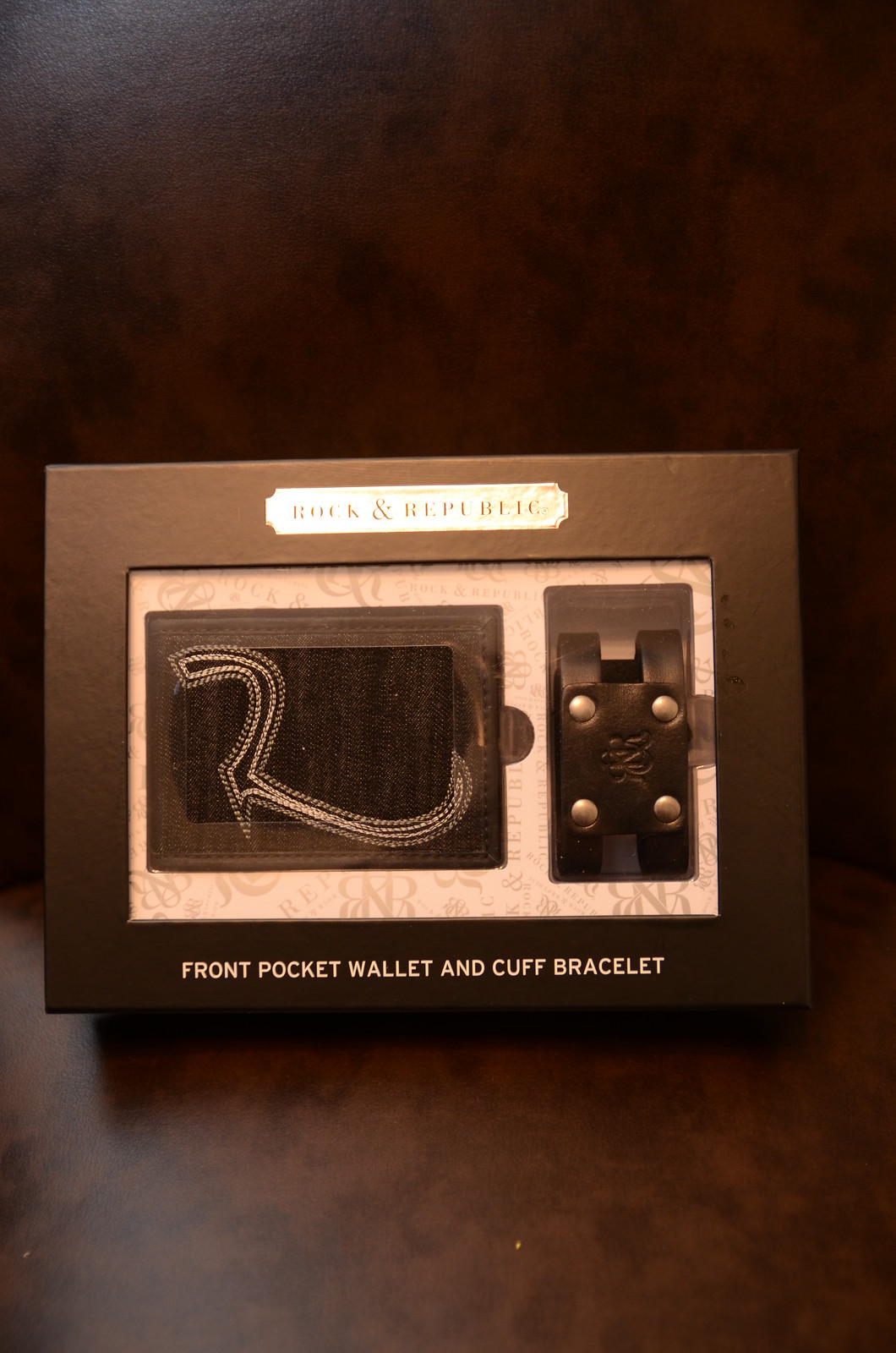The image is a color photograph in portrait orientation, showcasing a rectangular product box with a clear window displaying a brown leather front pocket wallet and a matching cuff bracelet. The box, labeled with the brand name "Rock and Republic," is positioned on a dark brown surface, likely a wooden table, and features a patterned beige and tan design around the displayed items. The wallet is adorned with an intricate, ornate swirl design and metal studs, giving it a Western feel. The cuff bracelet, also leather with similar metal details, is placed upright to the right of the wallet. The white text beneath the items reads "Front Pocket Wallet and Cuff Bracelet," clearly indicating the products inside. The background of the image is a dark gradient, highlighting the box in the center. The photograph adheres to the style of Photographic Representationalism, focusing on realism and detailed product presentation.